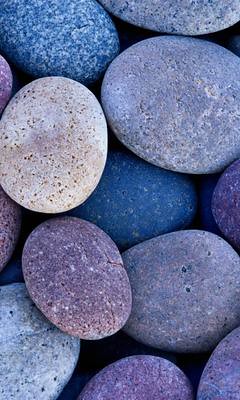The image features a vertically cropped collection of round and oval-shaped stones, meticulously arranged to create a visually striking, almost artistic display. The stones, appearing as a cohesive group, vary greatly in color, presenting a spectrum of hues that includes chalky whites, light and medium blues, brownish yellows, rustic reds, and speckled white and blue. Some stones even exhibit purples and other rare, vibrant shades not commonly found in nature, suggesting either natural weathering processes or deliberate dyeing. The overall composition, with its unique array of colors and perfectly rounded stones, gives the impression of an intentionally designed piece of art.